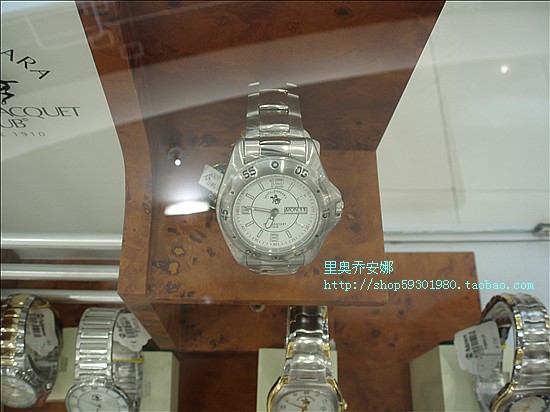This image features a meticulous display case of watches. On the left side of the display, a whiteboard is visible with black writing, which reads "Jaquette 1910". The bottom section showcases an array of elegant timepieces. 

On the far left, there is a silver and gold watch with a white face, accompanied by a white tag bearing black writing. Adjacent to it is an all-silver watch featuring a white face. Next in line is a silver watch with gold trimming on the outside and a white face. Positioned at the bottom right is another watch, silver with gold edges and a white face. 

At the top of this section, an all-silver watch with a white face is displayed on a brown shelf. Additionally, there is a green-colored website link in the image: http://shop59301980.taobao.com.